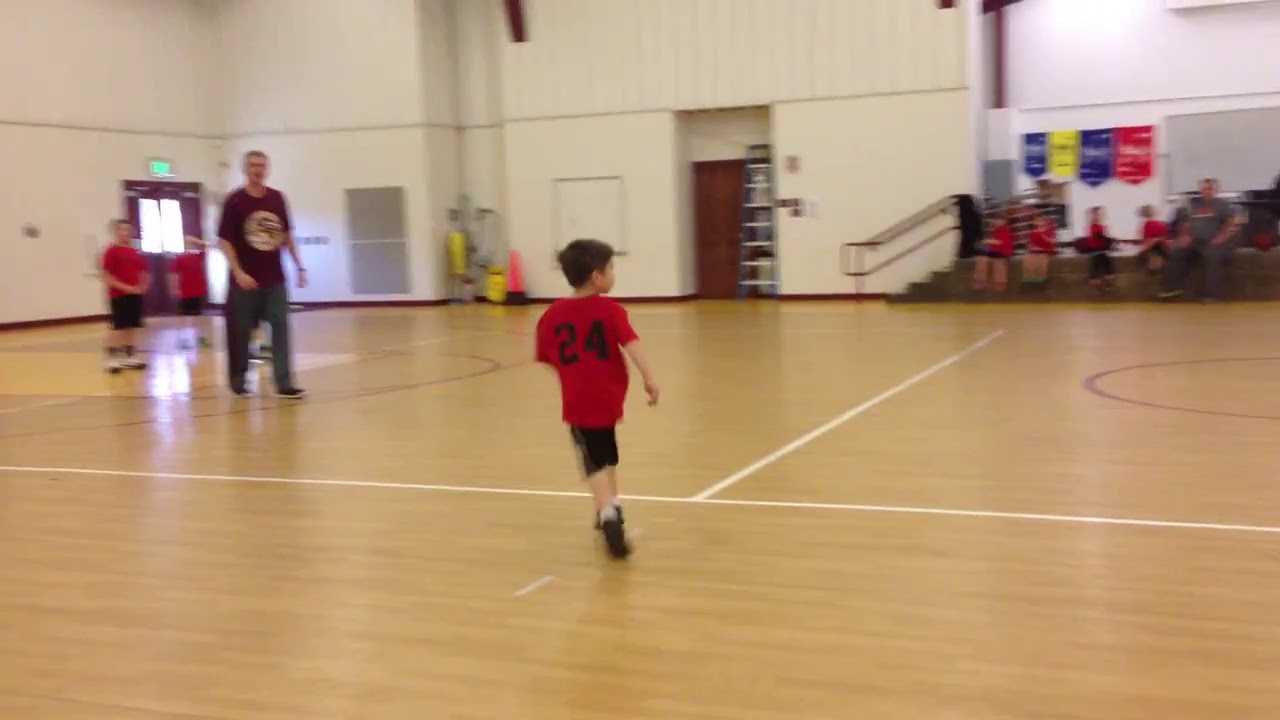The image captures a vibrant scene in a large, indoor gymnasium with white walls and honey oak wood flooring, marked clearly as a basketball court with various lines and circles. At the center, a young boy, around four or five years old, stands facing away from the viewer. He is dressed in a red t-shirt emblazoned with the black number 24, black shorts, and black sneakers. His attention is directed towards the right side where people are seated on the bleachers, possibly watching a game. To his left, an adult man dressed in a dark shirt displaying a circular logo and dark pants seems to be looking at him. Behind this man, two other boys, similarly dressed in red shirts and black shorts, stand in the end zone of the court. The backdrop includes colorful flags hanging on the walls and a door with a green exit sign above it. The photograph, which appears slightly blurred due to motion, captures a slice of dynamic activity within a realistic, representational style, reminiscent of a freeze-frame from a video.